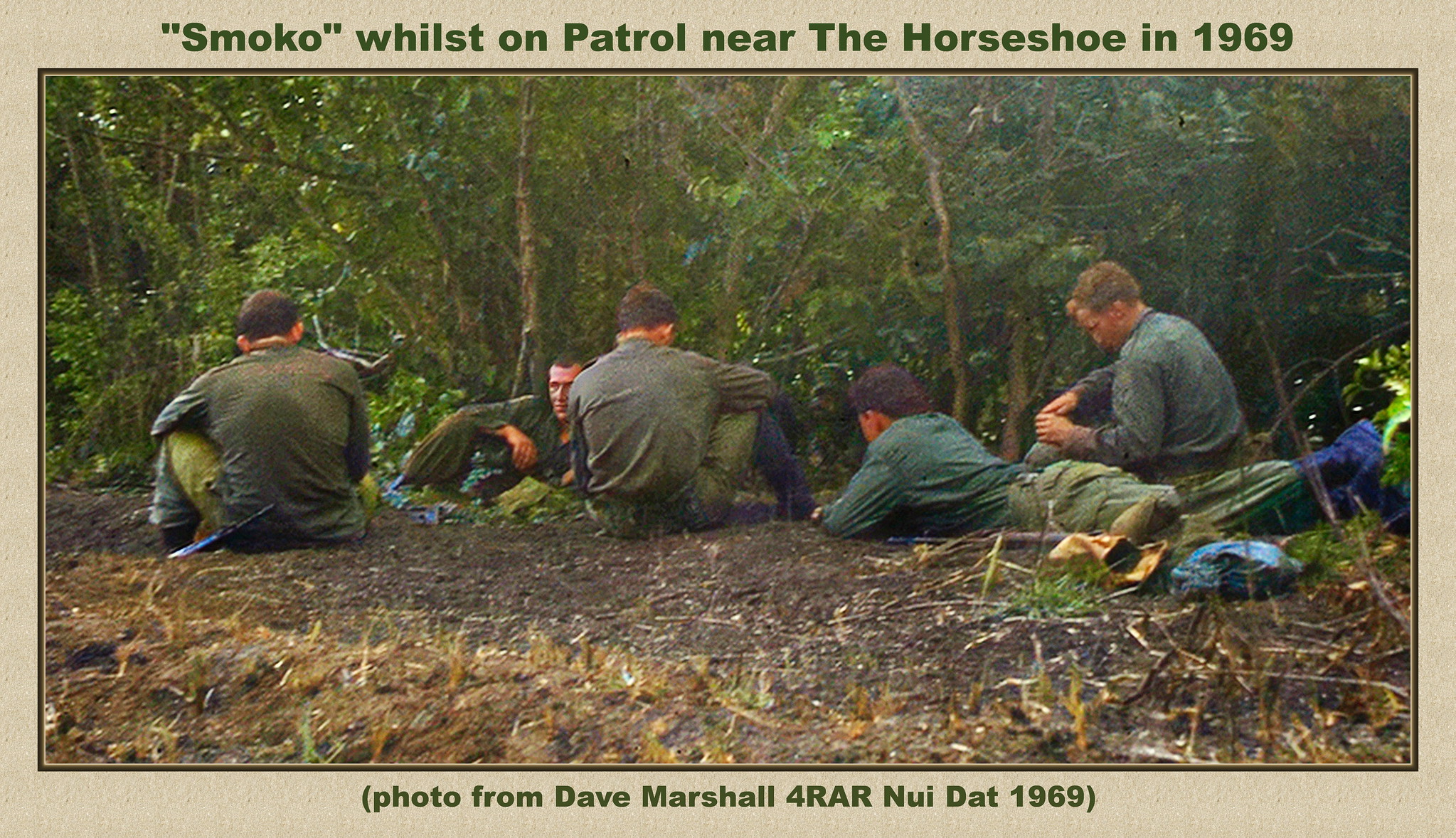This detailed color photograph from 1969, contributed by Dave Marshall for RAR Neuidat, captures a scene titled “Smoko” Wilson Patrol near the Horseshoe. The landscape picture is bordered in a grayish, creamish, greenish hue with green text at the top. At the bottom, additional text notes its source. The image features five men, presumably military personnel, resting on the earthy ground that is dotted with dead grass. The background is filled with dense foliage and trees. The men, all with dark hair and clad in dark green shirts paired with lighter green pants, are arranged in various relaxed postures - three seated and two lying down on the forest floor. Off to the right, a splash of color from potential gear or clothing adds to the scene's authenticity. This photograph eloquently documents a moment of reprieve for these men clad in green uniforms during their patrol in a forested area.